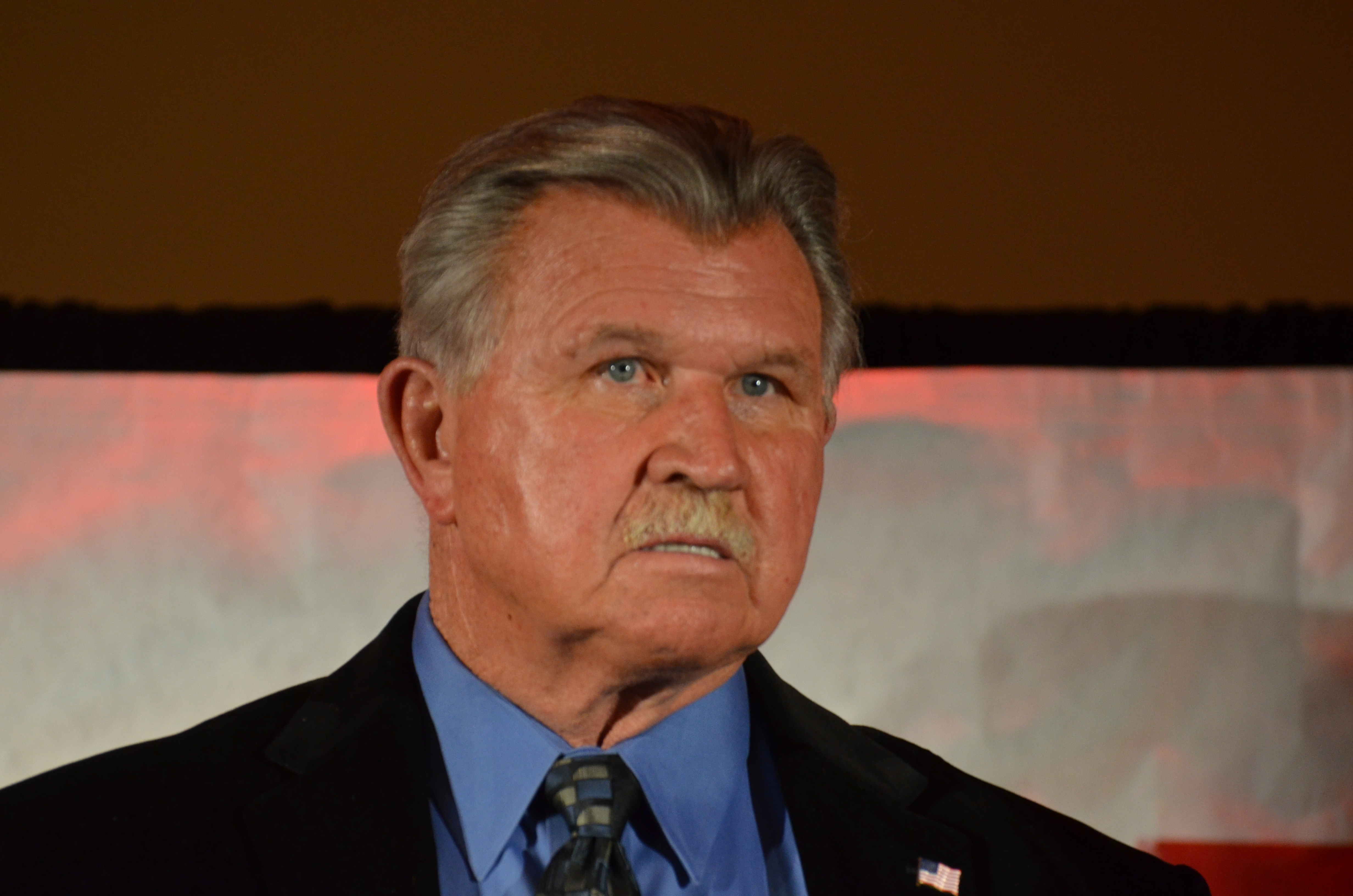The photograph depicts an older, light-skinned man, likely in his late 60s to early 70s, who is instantly recognizable as a football coach, although his name escapes memory. He stands in front of a brown-colored background that features a black horizontal stripe and a multi-colored design with shades of pink, orange, and green. The man has well-cropped, light brown hair with streaks of gray, forming a V on his forehead. His face, with visible wrinkles and a heavy-set nose, sports a grayed mustache. His piercing blue eyes and fierce expression suggest a moment of intense emotion, possibly agitation. He wears a dark blue or black suit jacket adorned with a USA pin on the right shoulder, a blue collared shirt, and a tie that is gray with a blue square pattern.